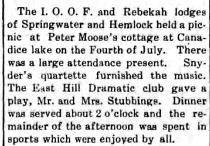The image features a newspaper clipping announcing a 4th of July picnic hosted by the IOOF and Rebecca Lodges of Springwater and Hemlock at Peter Moose's Cottage at Cannadice Lake. The clipping details that the event had a large attendance, with music provided by Snyder's Quartet and a play performed by the East Hill Dramatic Club. Mr. and Mrs. Stewbridge hosted dinner around two o'clock, followed by an afternoon of enjoyable sports activities. The image background is white, with black text centrally aligned and flanked by thin vertical black lines on both sides, giving it a structured appearance.